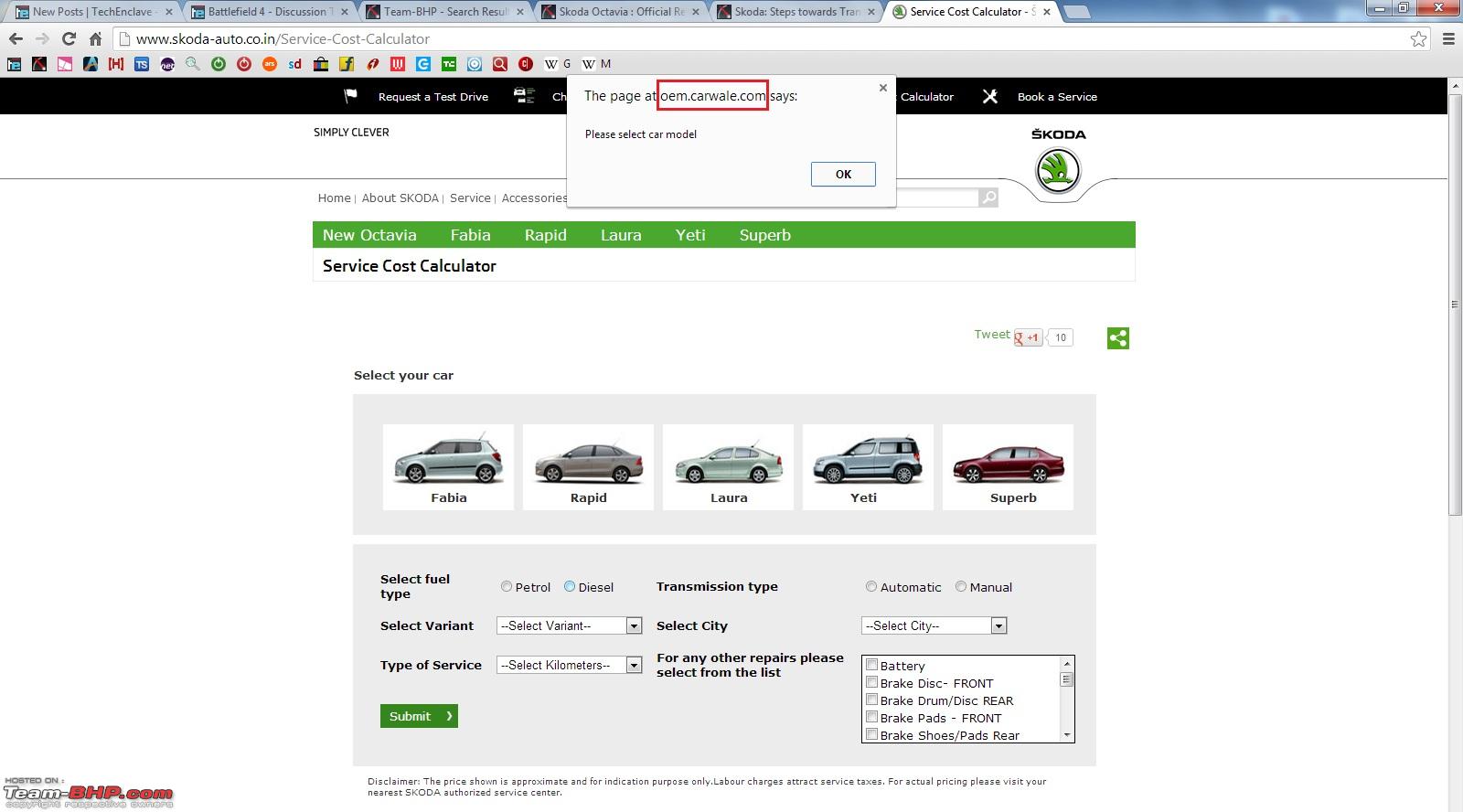Screenshot with a white background, displaying a browser window with six open tabs. The focus is on a website with a white pop-up box at the center of the page. The website is highlighted with a blue rectangle and prompts users to "Please select car model." 

At the top, the site is branded as "Simply Clever Škoda," showcasing various car models including the New Octavia, Fabia, Rapid, Laura, Yeti, and Superb. The interface includes a "Service Cost Calculator" and multiple selection options, such as:

- **Select your car**: Options listed are Fabia, Rapid, Laura, Yeti, Superb.
- **Select fuel type**: Two radio buttons for Petrol and Diesel, with Diesel currently selected and shaded blue.
- **Transmission type**: Choices between Automatic and Manual.
- **Select variant** and **Select city**: Both have drop-down selection boxes.
- **Type of service**: Includes a box to select kilometers.
- For additional repairs, a box prompts users to select from a list.

The pop-up box prominently features the details and selection options, ensuring users can easily navigate and complete their service cost calculations.